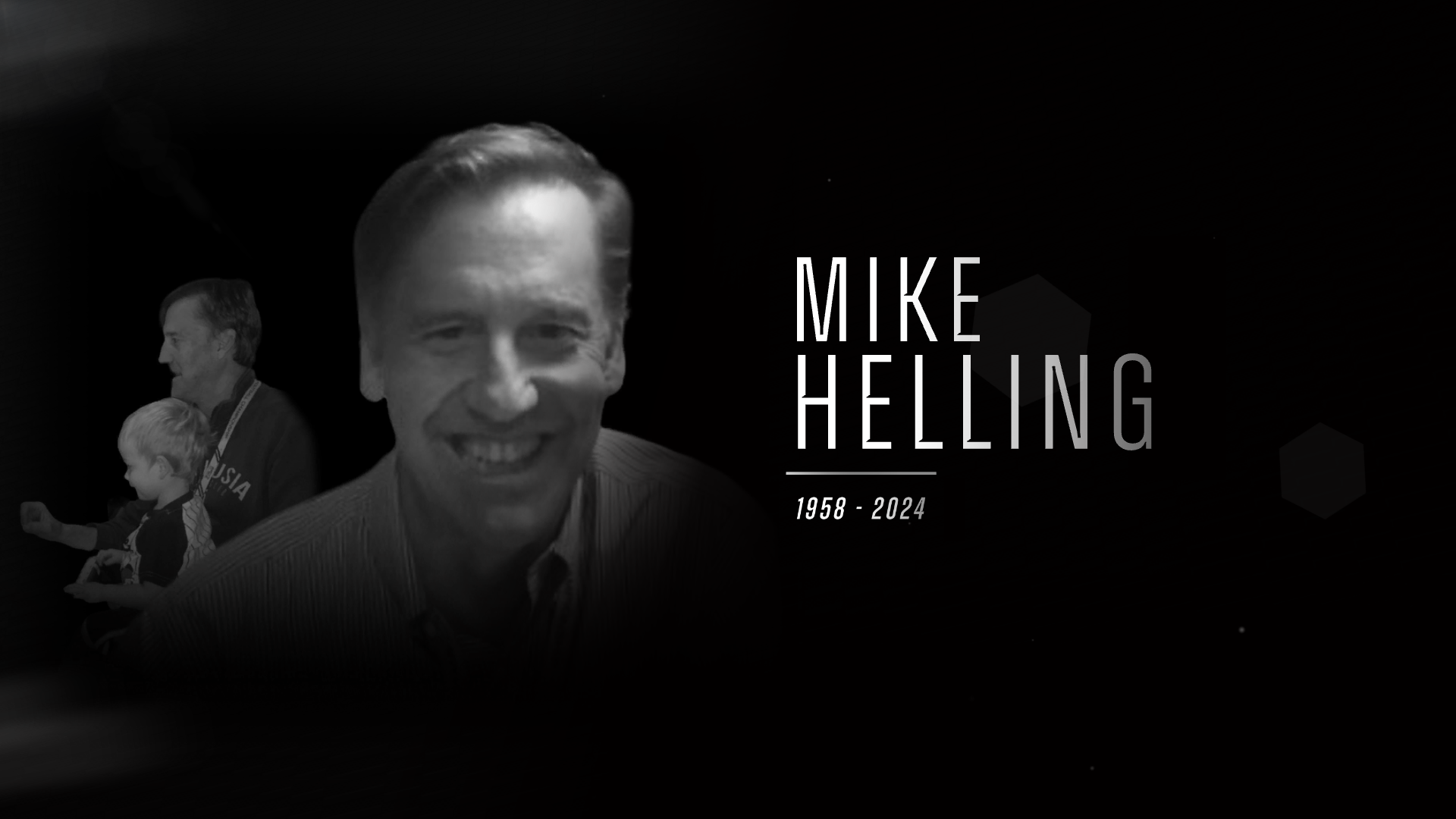The image is a black and white memorial banner featuring the late Mike Helling, with the text "Mike Helling, 1958-2024" in white font against a black background. The banner prominently displays two photos of Mike: the main photo to the right shows him smiling directly at the camera while wearing a suit, his face warmly illuminated despite the low quality of the image. To the left, there is a secondary image, slightly faded, of Mike seen in profile, casually dressed in a polo shirt with a lanyard, with a small child on his lap, both seemingly engaged in an activity. This simple yet poignant design likely created by his family or as part of a larger commemorative video, captures moments of happiness and intimacy, reflecting a tribute to his life and legacy.